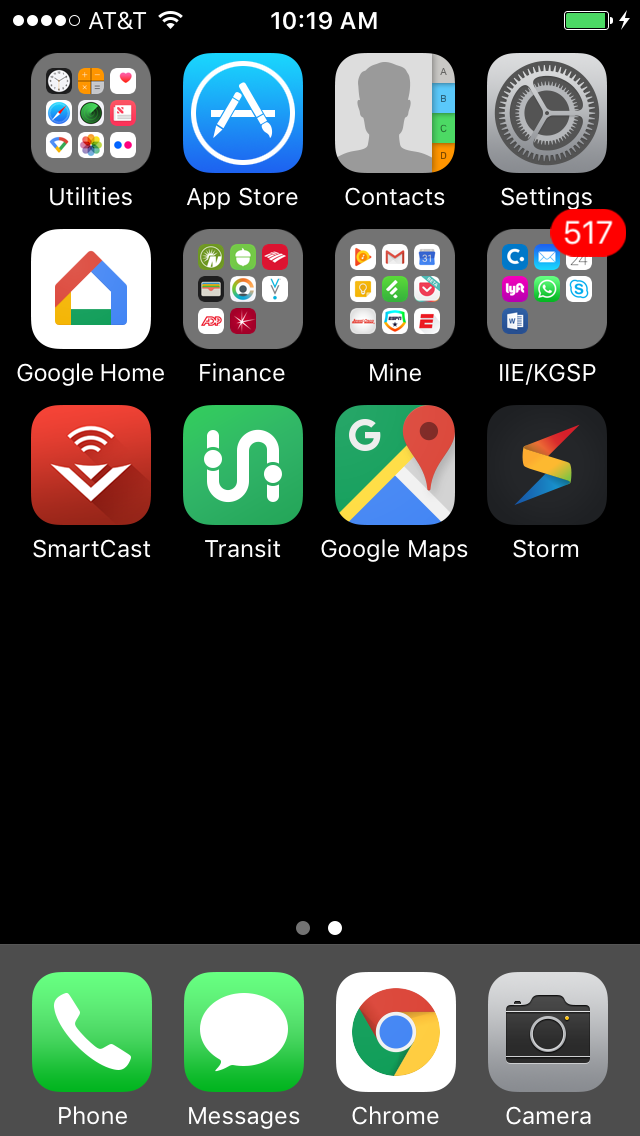The image depicts the main homepage screen of an iPhone. In the upper right-hand corner, there are five circular icons: the first four are filled with white, and the fifth is an outlined white circle. Next to these circles, in bold white letters, it says "AT&T." Following that, there's a Wi-Fi icon consisting of three solid white curved lines, indicating a strong Wi-Fi connection. The time displayed in the center is "10:19 AM" in capital letters. To the right, there's a battery icon outlined in white, mostly filled with green, suggesting a mostly charged battery. Inside the battery icon, there's a white lightning bolt, indicating the iPhone is currently charging. The background wallpaper of the screen is solid black.

At the bottom of the screen, there's a gray rectangle containing four app icons. The first two icons are green: the first one features a white phone icon with the label "Phone," and the second one shows a white chat bubble icon labeled "Messages." The third icon is white with a multicolored circle (red, yellow, green, and blue) inside, labeled "Chrome." The last icon is gray with a darker gray camera icon and an orange dot, labeled "Camera."

Above these, there are 12 additional app icons arranged in the following order from the bottom left-hand side: SmartCast, Transit, Google Maps, Storm, Google Home, Finance, Mine, IIE/KGSP, Utilities, Apple Store, Contacts, and Settings.